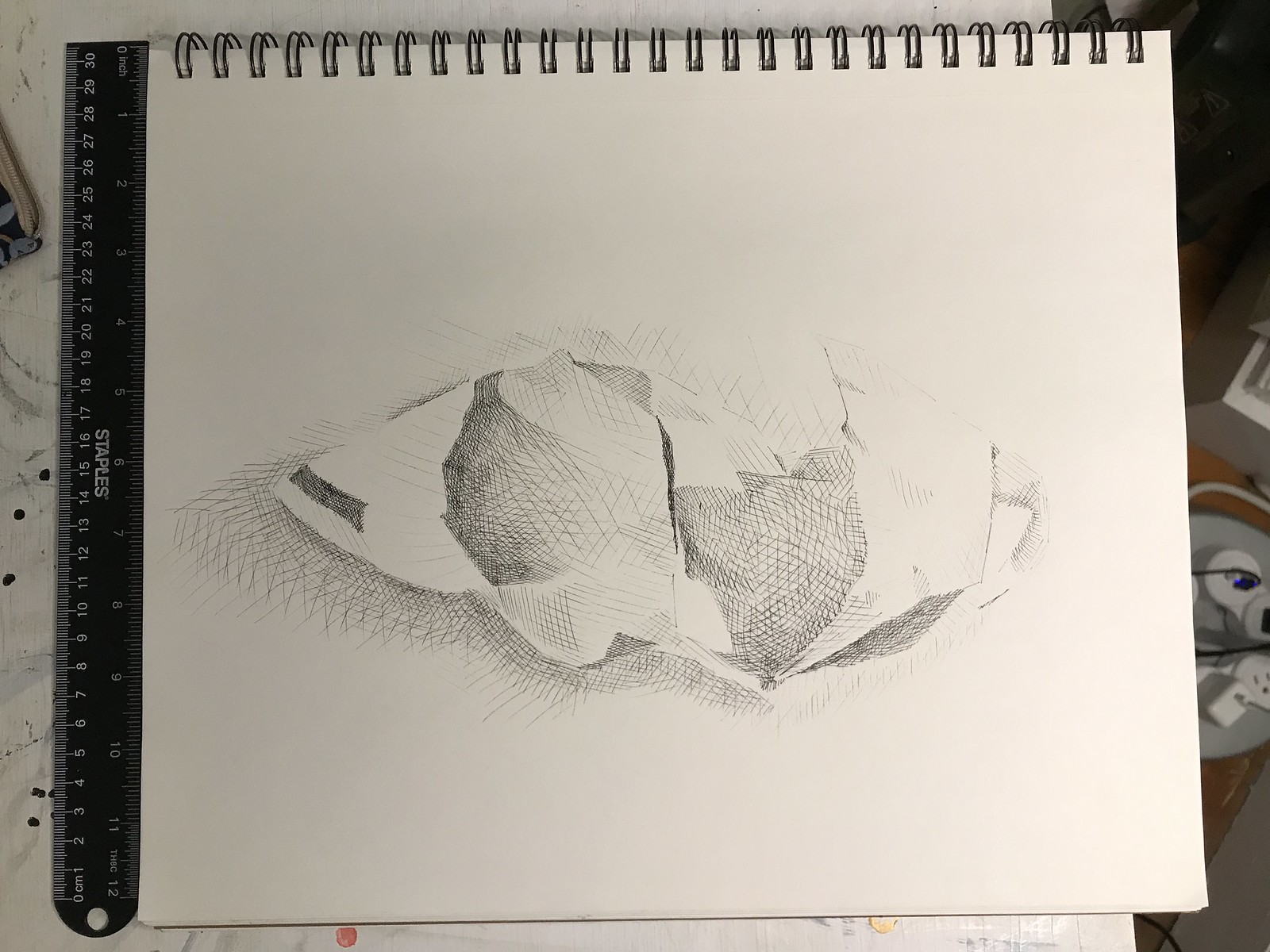This image captures a detailed pencil sketch of a fish, nestled on a white sheet within a sideways-turned sketchbook. The metal rings of the sketchbook are at the top of the image, and a black metal ruler rests along the bottom right edge. On the left side, the sketchbook sits on a white surface, with a carpeted floor visible in the background. The top-down perspective highlights the intricate pencil work, portraying the fish with dark, hatched areas to depict its distinct markings. The fish appears to be an orange and black variety commonly found in ponds, and its tail is sketched to the side, suggesting the motion of it flopping on the ground.